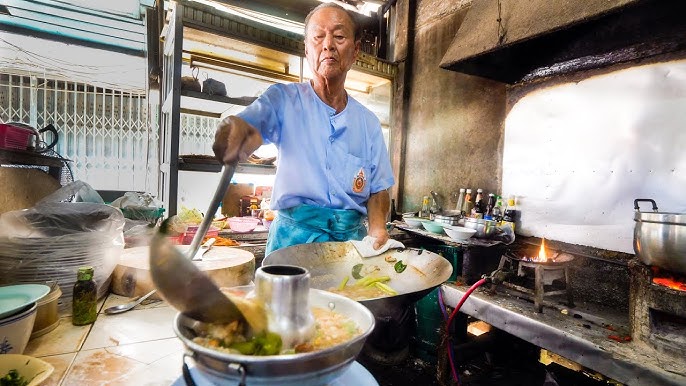In this vivid color photograph, an elderly Chinese chef, clad in a light blue button-down shirt and a greenish-blue apron, stands in the bustling, industrial-style kitchen of an urban restaurant. The kitchen is set up in a rudimentary fashion, with various utensils, plates, bowls, and bottles of sauce scattered around. The chef, approximately 70 years old, is centrally framed in the image, deeply focused on his culinary task. He is ladling a soup, filled with green vegetables that might include peppers, into a metal bowl that features a distinctive silver hollow tube in the center. The ladle, thrust toward the camera, creates a dynamic, almost 3D effect. In his left hand, the chef holds a wok partially filled with food, using a white towel for grip. Behind him, the kitchen counters are cluttered with more cooking equipment, including a gas burner cooktop, a steel round container over a fire, and various bottles of spices and condiments. The backdrop showcases a metal vent hood and, further back, glass windows revealing a cloudy urban skyline. The photograph captures the essence of a traditional, busy kitchen scene with remarkable realism.